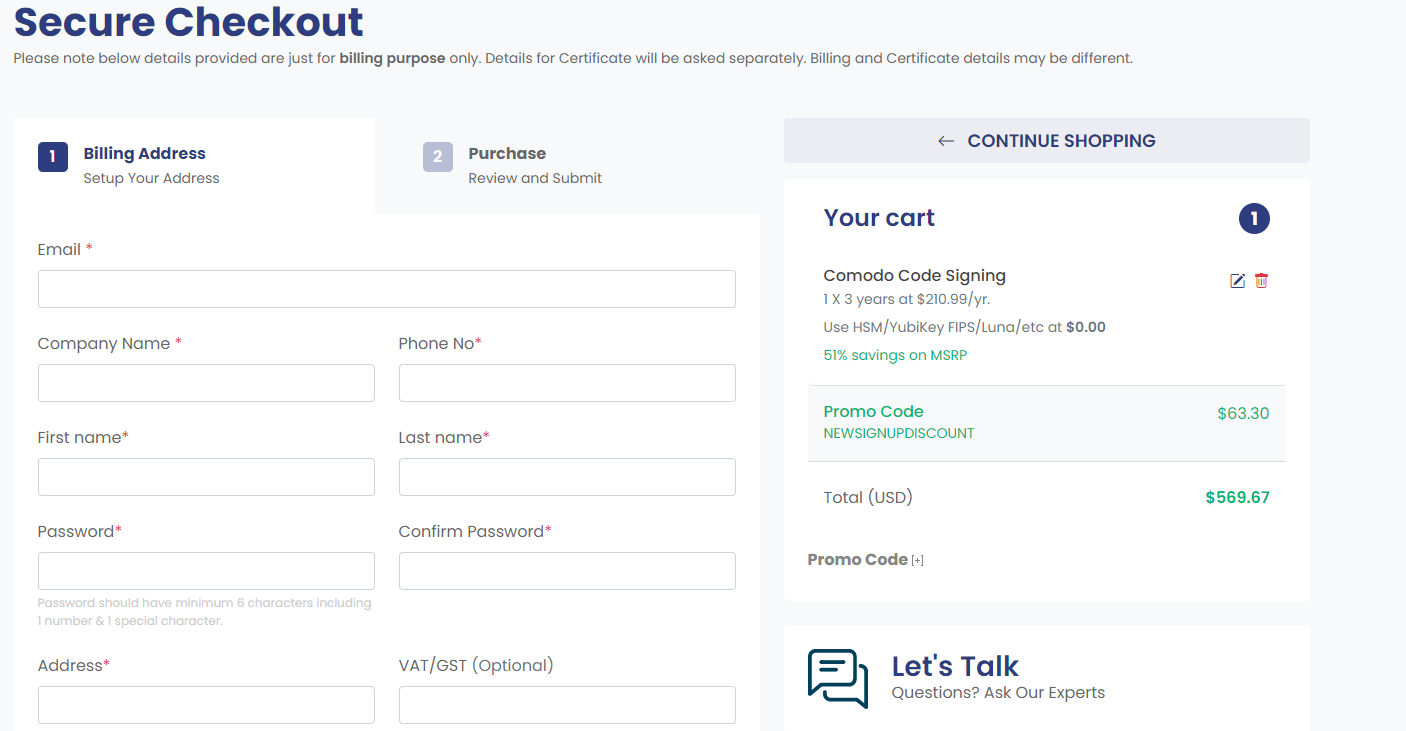This digital screenshot displays the secure checkout page for purchasing a service. The page is structured to collect detailed billing information, which is strictly for invoicing purposes, with separate fields for certificate information to be entered later. 

Users are prompted to enter their billing address, email address, company name, phone number, first name, last name, and to create and confirm a password that meets specified security criteria (minimum six characters, including at least one number and one special character). 

The form also includes a field for an optional VAT/ZST number. 

Additionally, the cart section shows a selected item: "Komodo Code Signing" for a period of three years, priced at $210.99 per year, reflecting a 51% savings off the MSRP. There is also an option to enter a promo code, and a mention of a new sign-up discount.